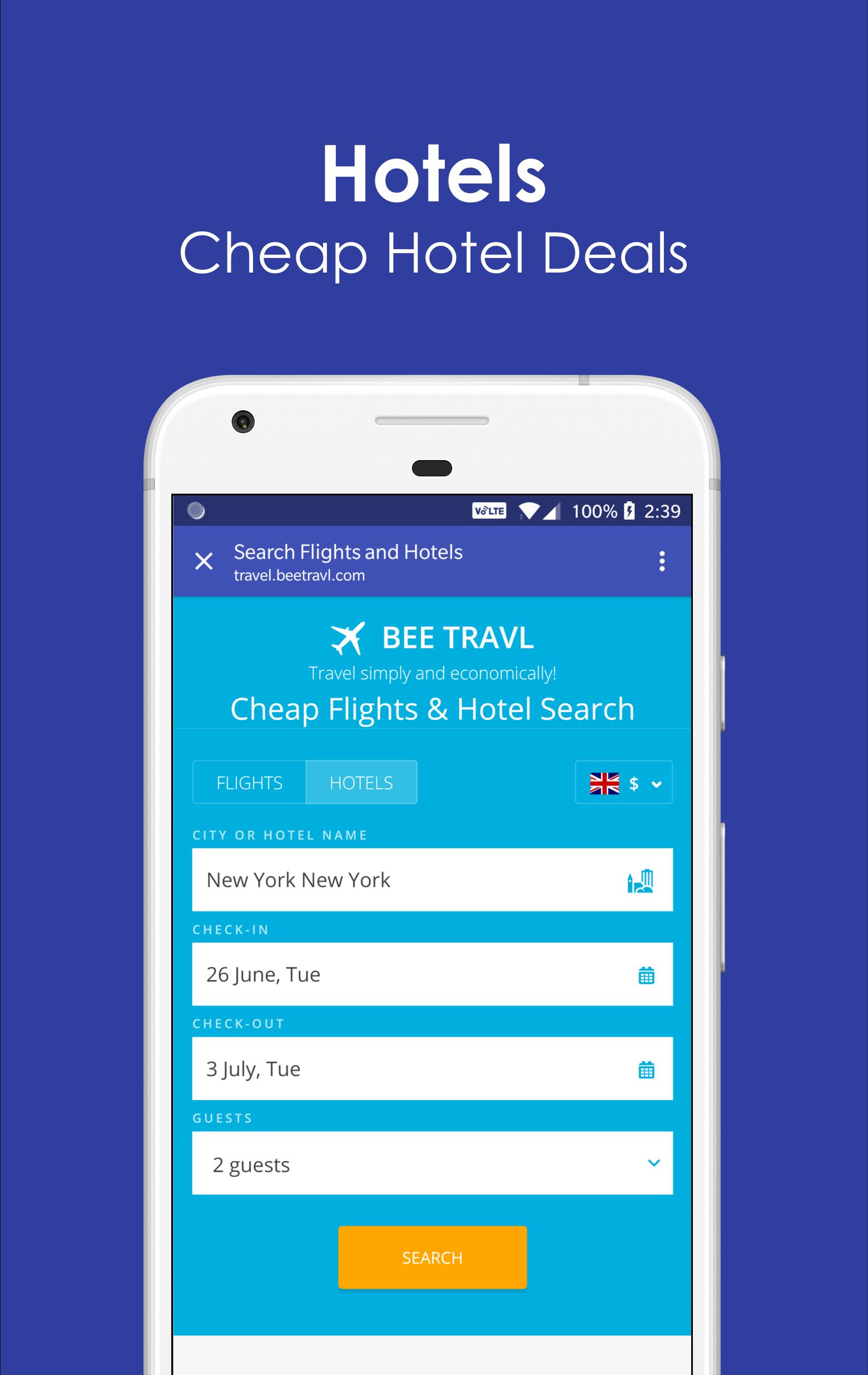The digital image showcases a smartphone against a bluish-purple background. At the top center, bolded white text reads "Hotels," with smaller, thinner text below it stating "Cheap Hotel Deals." The smartphone features a white bezel, thicker at the top, and houses a black lens on the top left, a light gray speaker at the top center, and a black pill-shaped element beneath the speaker.

The phone's simulated screen displays a mobile page, beginning with a dark blue header featuring white icons on the right. Below this is a lighter blue header containing a white 'X' on the left and two lines of text to the right. The larger text says "Search Flights and Hotels," and below it reads "travel.btravel.com," with "B-Travel" spelled B-E-E-T-R-A-V-L. On the far right of this header, there are three vertical white dots.

The main body of the page has an aqua blue background. At the top center is large, all-caps white text reading "B-Travel," accompanied by a white plane icon to the left, angled upwards at 45 degrees. Below this, a line of small white text says, "Travel Simply and Economically!" followed by larger white text stating "Cheap Flights and Hotels Search."